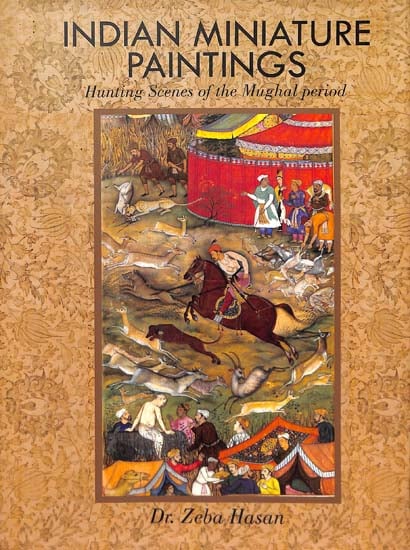The photo features a book titled "Indian Miniature Paintings: Hunting Scenes of the Mughal Period" by Dr. Ziba Hassan. The book cover is adorned with a tan background featuring an intricate pattern. At the center of the cover, there is a vibrant and detailed illustration characteristic of Indian miniature painting from the Mughal period. The scene depicts a hunting expedition, showcasing various figures including a hunter on horseback, a dog, and wild animals that could be a goat or an elk. The foreground features what appears to be royalty or affluent individuals, indicative of the period's depiction of societal hierarchies and leisure activities. The brightly colored composition and meticulous detail reflect the richness and finesse typical of miniature paintings, making the cover itself a work of art reminiscent of museum exhibits.